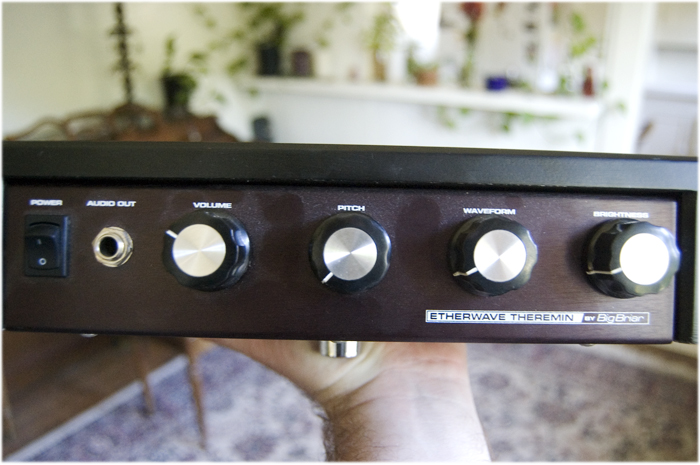This image shows a close-up of the front of an Etherwave Theremin, a unique musical instrument known for its eerie sounds. The theremin is encased in a brown wooden box with a black top. Multiple black and white knobs, each with a distinctive white or metallic-looking circle in the middle and a black edge, adorn the device. On the left-hand side, there's a black on-off power switch clearly labeled "power," followed by an "audio out" port. To the right, there are successive knobs labeled "volume," "pitch," "waveform," and "brightness." In the lower right-hand corner, the text "EtherWave Theremin Big Briar" is prominently displayed. The image features a man's hand holding up the theremin, his arm emerging from the bottom of the frame. As a backdrop, you can see a living space with a wooden floor covered by a rug, various household items on a shelf, and some greenery, indicating the photo was taken in a domestic setting.